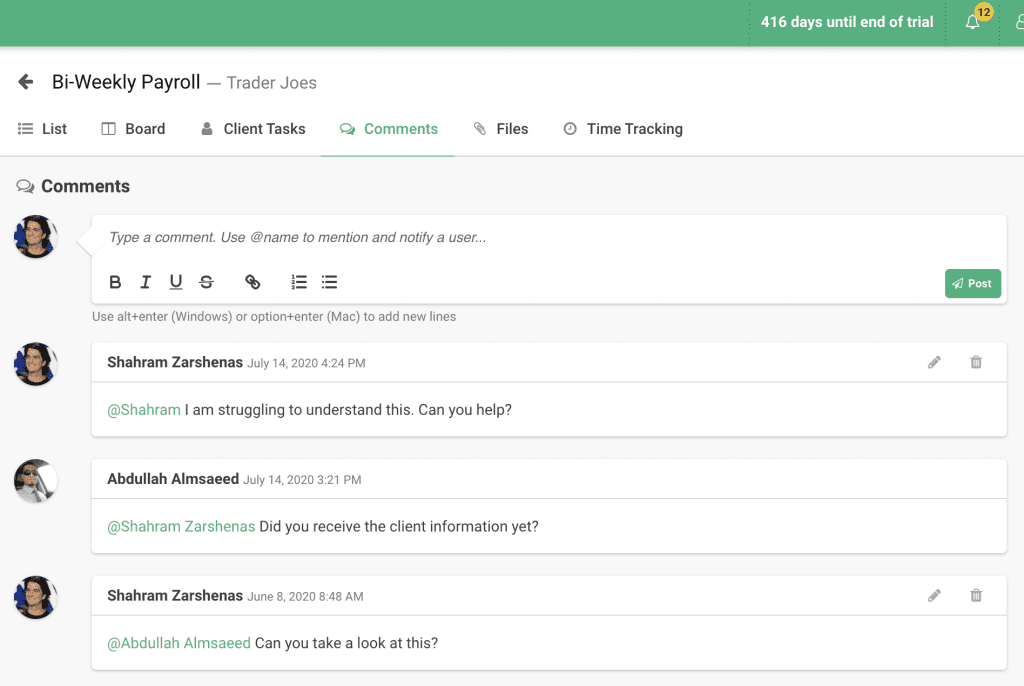The image shows a detailed screenshot of a work-related app, likely functioning as an employee portal for Trader Joe's. The top of the screenshot features a green navigation bar. On the right side of this bar, text reads "416 days until end of trial," accompanied by a bell icon indicating 12 notifications, and a partially visible profile icon. 

Directly below the green bar, there's a left-pointing arrow and bold text reading "Bi-weekly Payroll" with smaller, grey text below it specifying "Trader Joe's," suggesting this portal serves Trader Joe's employees.

Below this title, a vertical menu lists various sections: list, board, client, tasks, comments, files, and time tracking. The "comments" section is highlighted in green, showing that it is currently active. 

On the main part of the page, the word "Comments" with an accompanying icon is prominently displayed. Below, a messaging interface shows a conversation, depicted in four sections, between two individuals. Three messages feature an image of one man, while the third has a different man's picture. The conversation appears as follows:

- **First Message (bottom):** "Can you add the person or tag the person saying can you take a look at this."
- **Second Message:** "Did you receive client information yet."
- **Third Message:** "I am struggling to understand this, can you help."
- **Fourth Message (top):** A blank input bar ready for the next response.

This detailed view highlights the interactive elements and structured interface of the Trader Joe's employee portal, showcasing both navigational features and user communication.